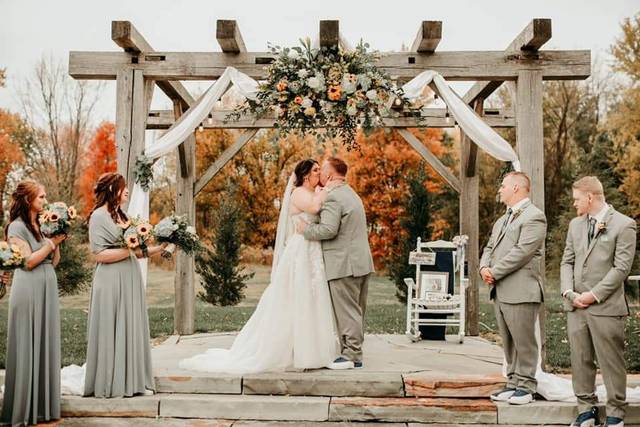A beautifully detailed photograph depicts a couple sharing a kiss during their wedding ceremony, set against a picturesque outdoor backdrop. The couple stands beneath an elegant wooden canopy adorned with white curtains on either side and an arrangement of colorful flowers at its peak. The bride, positioned on the left, dons a stunning white dress and the groom, on the right, is dressed in a gray suit and gray pants. The setting suggests a fall wedding, as evidenced by the changing colors of the leaves on the green and brown trees in the background, and the bridesmaids to the left of the bride, who are wearing shawls over their dresses, presumably due to the chilly weather. Two men stand to the right of the groom, dressed similarly to him, and two bridesmaids, holding bundles of yellow flowers, stand to the left. The overall scene exudes elegance and intimacy, capturing a joyous moment amidst the natural beauty of the season.